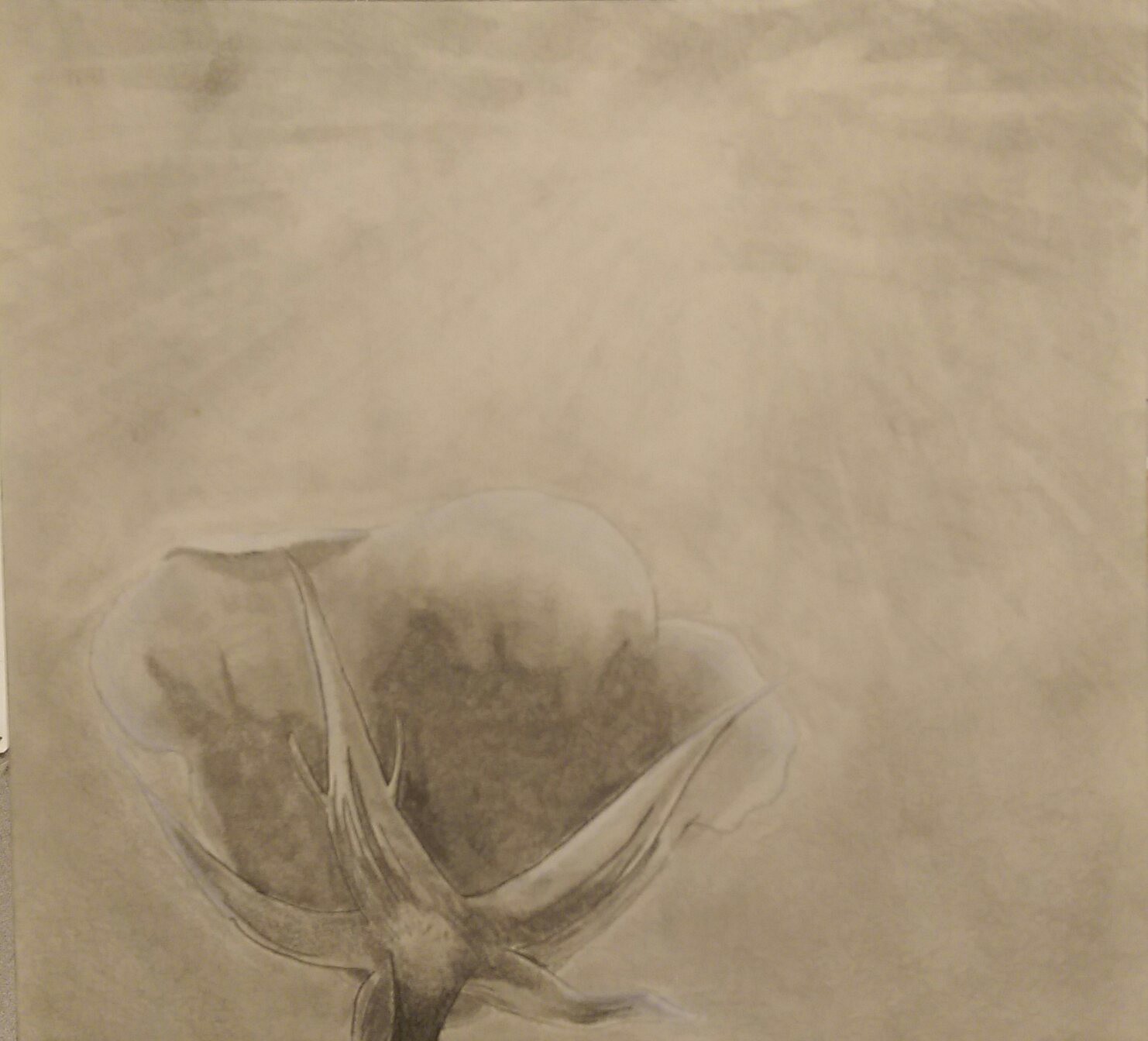The image features a intricately detailed pencil sketch of a single rose, prominently situated in the bottom-left corner of an off-white piece of paper. The rose's stem extends upward, culminating in three well-defined, textured petals which exhibit a graceful, three-dimensional appearance. The petals and stem are rendered in shades of gray, black, and tan, adding to the organic realism of the drawing. The background is filled with broad, consistent strokes of gray shading that converge towards a point roughly 10% down from the top and 60% over from the left, giving a sense of focused light, albeit in an abstract, not sharply defined manner. Overall, the drawing exudes a sense of depth and texture, resembling something made from suede or leather, and stands out against the otherwise plain background.